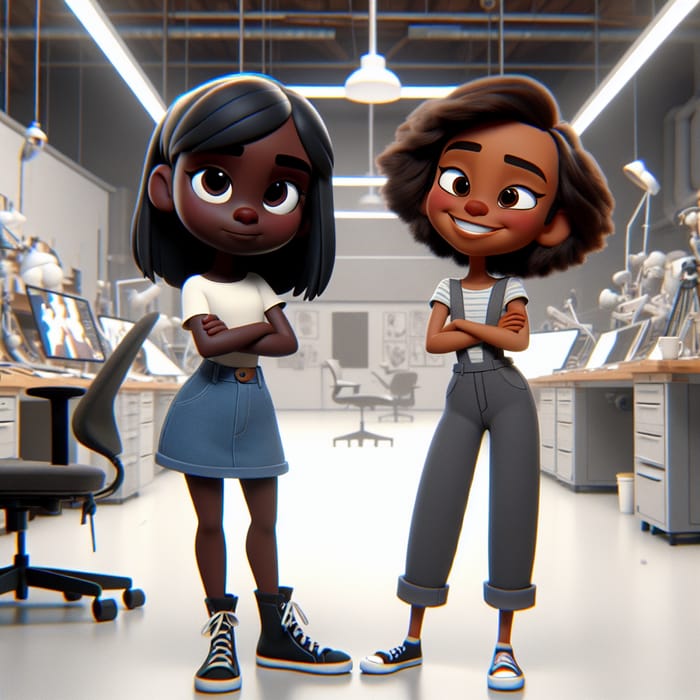This image is a computer-generated drawing of two young women of African descent, standing with their arms crossed and smiling directly at the viewer. Both appear to be in their late teens or early twenties and are dressed casually. The woman on the left has shoulder-length black hair, a white top, a blue denim skirt, and black shoes. The woman on the right, who has a shorter bob haircut, is dressed in a grey jumpsuit with the pants rolled up at the ends, black sneakers, and a white striped shirt. They are depicted in a modern office or laboratory setting, with computer screens, desk chairs, and various pieces of equipment in the background, all situated on a white floor. The overall ambiance of the scene suggests a high-tech, engineering, or programming environment.